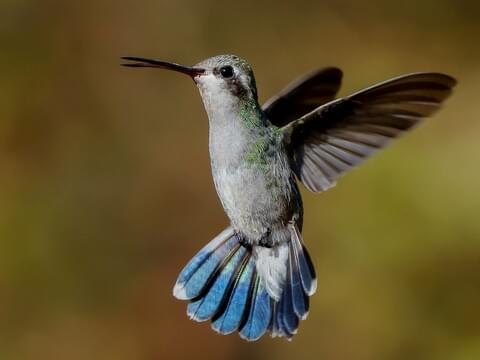This professional close-up photograph captures a stunning broad-billed hummingbird in mid-flight, sharply focused against a beautifully blurred, yellow-green background with hints of orange. The hummingbird, primarily situated at the center of the image, exhibits intricate details in its plumage and anatomy. Its long, slender beak, which appears to separate into two pieces, is colored in dark black with brown undertones. The bird's eye is also a striking dark black, and it faces towards the left of the image.

The bird's head is adorned with brownish feathers transitioning into a vibrant green across its back. Its chest and body are covered in pristine white feathers, adding a stark contrast to its colorful palette. The wings, expansive and dynamic in motion, showcase a blend of light green and brown feathers, with their size almost matching the length of the bird's body. 

The tail feathers are particularly captivating, with white bases transforming into tips of bright blue, accented with white edges. These tail feathers, numbering at least 10 to 15, display an array of beautiful shades including blue, white, yellow, and hints of black. This detailed and vivid representation of the broad-billed hummingbird, framed against a softly blurred backdrop, emphasizes its elegance and the intricate beauty of its feathers and form.